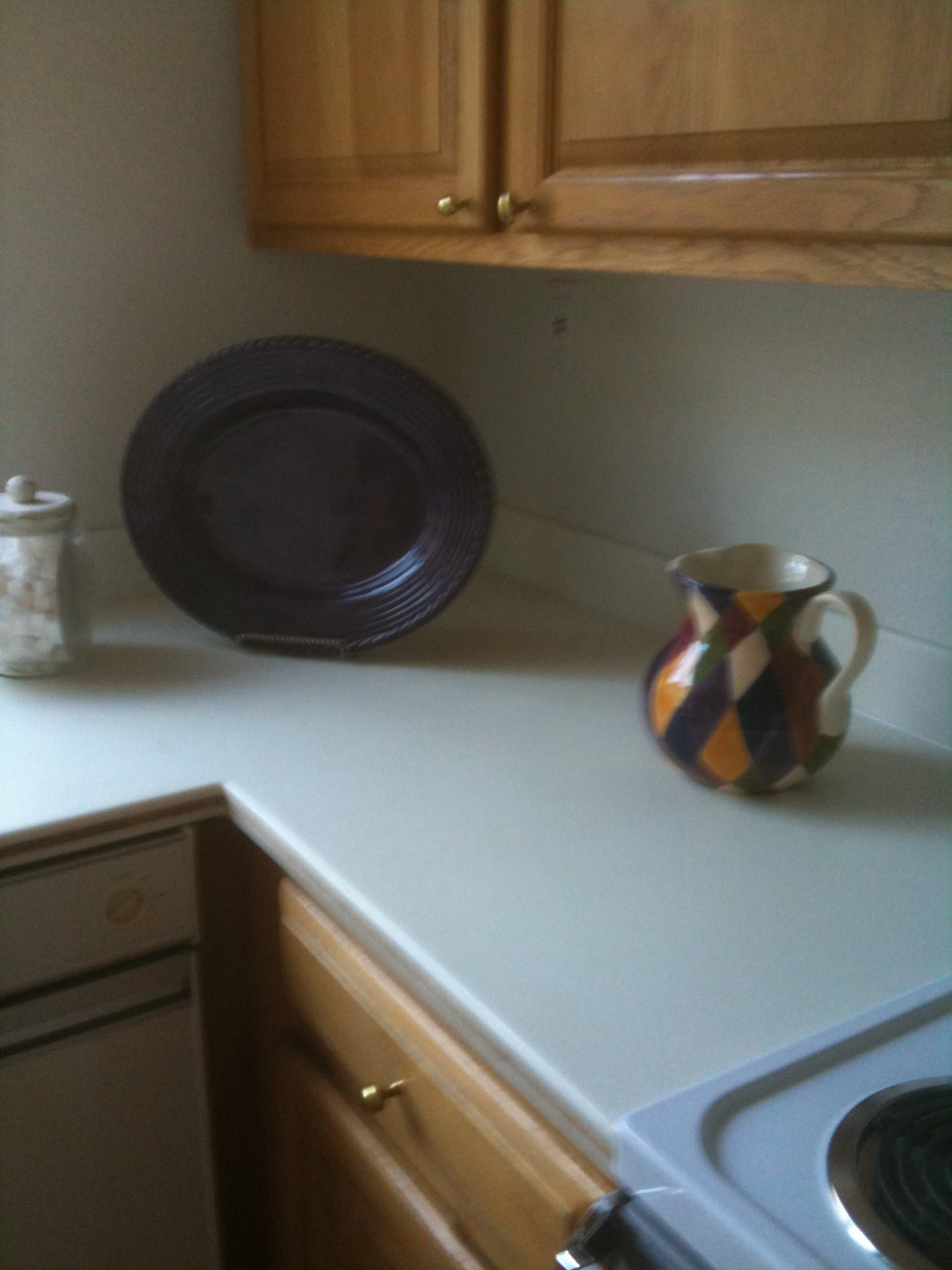This detailed photograph captures a well-organized corner of a kitchen. The off-white countertop is seen from an angled, top-down perspective, near a corner wall. A matching white backsplash complements the countertop. A round, dark plate, turned on its side, rests on a black plate rack. At the top of the image, the bottom edge of a wooden cabinet is visible, with gold-colored drawer pulls providing a touch of elegance.

In the lower right corner, part of a white stove is visible, showing a burner and the stove's front edge. On the countertop, slightly to the left, there's a white container with a lid—its contents indistinguishable—adding to the kitchen's neat appearance. Adjacent to the stove sits a small, decorative ceramic pitcher adorned with a brown, orange, and off-white checkered pattern. The pitcher’s handle is facing the stove.

On the bottom left, a lighter wood cabinet with matching gold-colored handles completes the scene, underpinning the kitchen's warm and cohesive design elements.